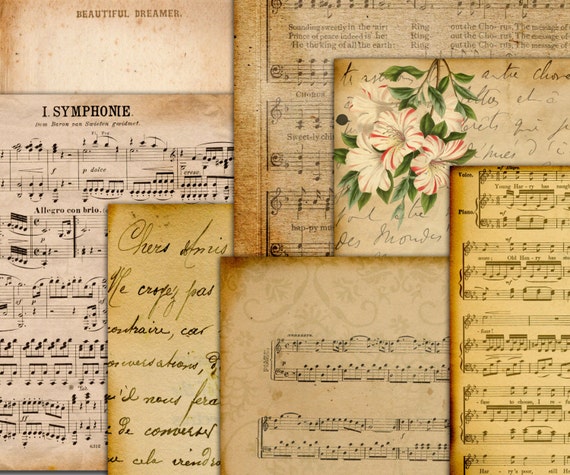The square image, devoid of discernible border or background, showcases an intricate arrangement of seven overlapping sheets of aged, brown, watermarked, and stained paper. Predominantly featuring sheet music, the most discernible titles include "Beautiful Dreamer" on the top left and "One Symphony" (or "iSymphony") directly beneath it. The music notes on these sheets cascade downwards, with "One Symphony" nearly reaching the bottom of the image. Handwritten notes intersperse the assembly, with one on the right partially covering the sheet below. Additionally, a handwritten note near the center-right is adorned with an image of red and white flowers. The overall arrangement subtly extends beyond the image's edges, enhancing the old, weathered charm of the layered papers.